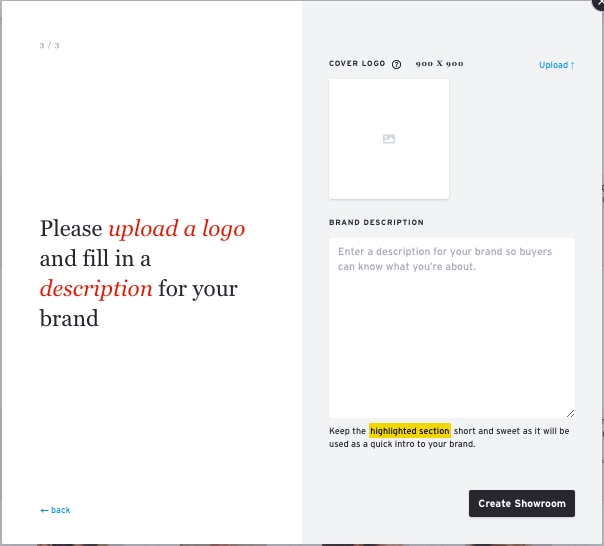This image is a screenshot of a webpage, specifically page 3 out of 3, from a website designed to help users build an advertisement or create a logo. The page layout is divided into a left and right section, with the left side featuring a white background and the right side a gray background.

On the left side, there is a prompt that reads, "Please now upload a logo and fill in a description for your brand." The words "upload a logo" and "description" are highlighted in red, while the rest of the text is in black.

The right side of the page includes an instruction that says, "Cover logo 900 by 900," accompanied by an upload button. This is where users are required to upload their logo. Below the upload area, there is space to type a brand description once the logo has been uploaded.

At the bottom of the page, there is a note advising users to, "Keep the highlighted section short and sweet as it will be used as a quick intro to your brand."

This is the final step (part 3 of 3) in the process, after which users will be able to create their own showroom, suggesting that this tool is designed for creating an online space to display and sell products.